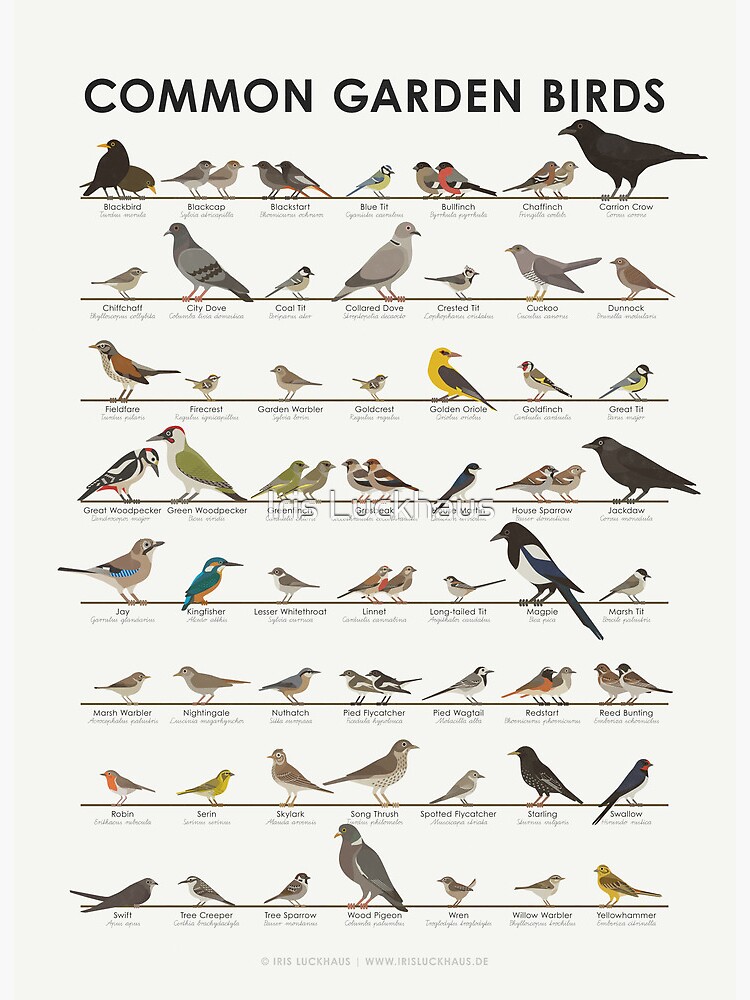The image is a full-color, vertically oriented poster titled "COMMON GARDEN BIRDS." Set against a white background, the poster is organized into 8 horizontal rows, each containing approximately 7 birds. Each bird is vividly illustrated in various colors, including black, yellow, green, brown, gray, and combinations thereof. Underneath each bird, their names are written in black text. The birds are listed alphabetically from the top left to the bottom right. The first row starts with birds like the Blackbird, Blackcap, and Blackstart, and it ends with Yellowhammer at the bottom. Notable bird types include Blackbirds, Kingfishers, Finches, and Wrens. In the middle of the poster, there is a watermark that reads "Iris Luckhouse."